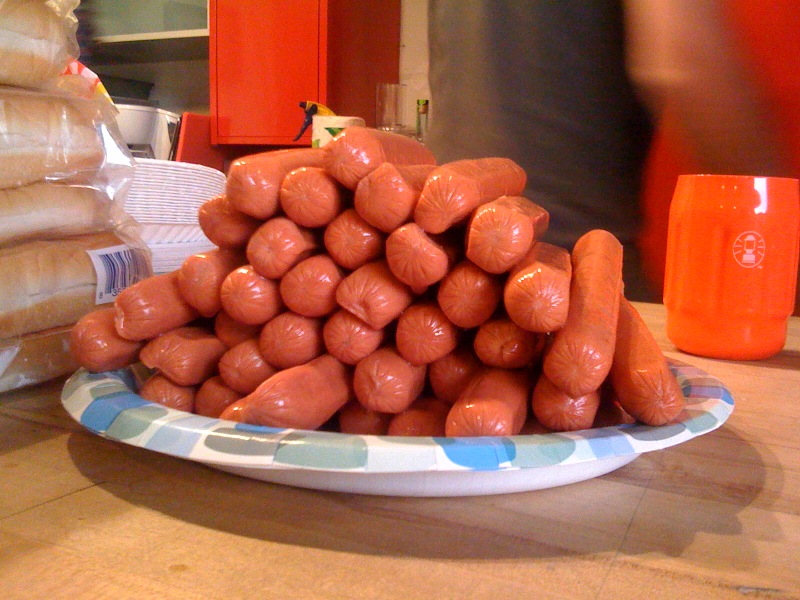The image shows a white paper plate adorned with blue and gray, or possibly green, dotted designs, brimming with an impressive stack of around two to three dozen uncooked hot dogs. The hot dogs, bright red in color, are piled into a somewhat haphazard pyramid shape, some falling or drooping. The plate rests on a wooden or butcher block laminate table, likely in a kitchen setting. To the left of the hot dogs, several packages of hot dog buns remain in their clear plastic packaging. An orange cup featuring a small white logo, possibly of a computer, sits to the right of the hot dogs. A stack of additional paper plates and red kitchen cupboards are visible in the background. The whole scene is bathed in indoor lighting, adding to the sense of a bustling food preparation area.